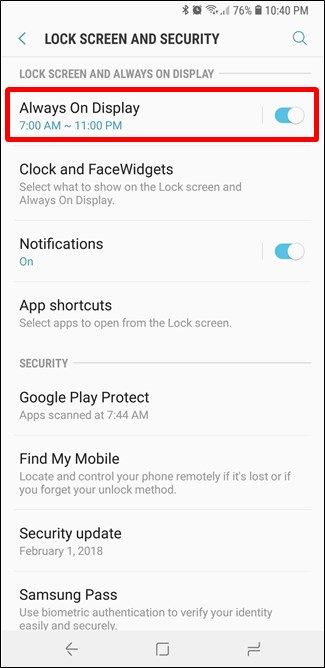This image captures a screenshot from a mobile phone's settings menu, with a focus on the "Lock Screen and Security" section. The background is white, and in the upper left corner, there are several status icons: a Bluetooth icon, an alarm clock icon, a Wi-Fi icon, a mobile signal icon, an indication of 76% battery life, a battery icon, and the time displayed as 10:40 PM.

Below this information, at the top of the settings menu, in black font, it says "Lock screen and security." To the left, there is a small left-pointing arrow, and to the right, a blue magnifying glass icon for search.

The next section, in gray font, reads "Lock screen and always on display." Just below, there is an entry for "Always On Display" from 7 AM to 11 PM, which has been circled in red, emphasizing its importance or relevance.

Following this, there is an option labeled "Clock and FaceWidgets" with a brief description: "Select what to show on the lock screen and always on display."

Below this, a "Notifications" toggle is visibly switched on, indicating notifications are enabled on the lock screen.

Next, there's an "App Shortcuts" option, allowing the user to select apps that can be opened directly from the lock menu screen.

Further down, under the "Security" section, there is mention of "Google Play Protect," indicating that apps were last scanned at 7:44 AM.

Finally, the "Find My Mobile" feature is noted, which allows the user to locate and control their phone remotely if it's lost or if they forget their unlock method.